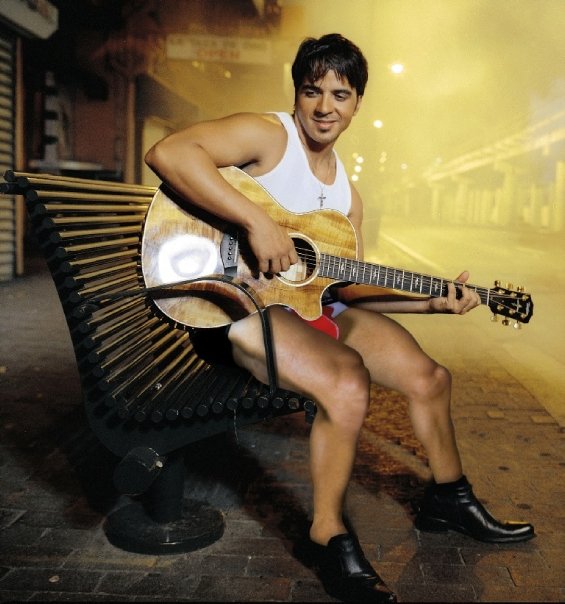The photograph features a young man with medium-length dark brown hair, seated on a black park bench, which is located on a dark brown brick pavement. He is playing a light brown guitar while smiling and looking down. The man is dressed in a white sleeveless t-shirt or tank top, adorned with a crucifix hanging from a chain around his neck. He is also wearing very short red and white shorts that reveal his muscular bare legs, accompanied by black dress shoes. The setting appears to be an empty small street at night, illuminated by streetlights, with blurry shops and signboards on either side. The overall image has a yellow tone, suggesting an aged or photoshopped look, and there is a smoky or dusky atmosphere in the background, contributing to its nostalgic feel.